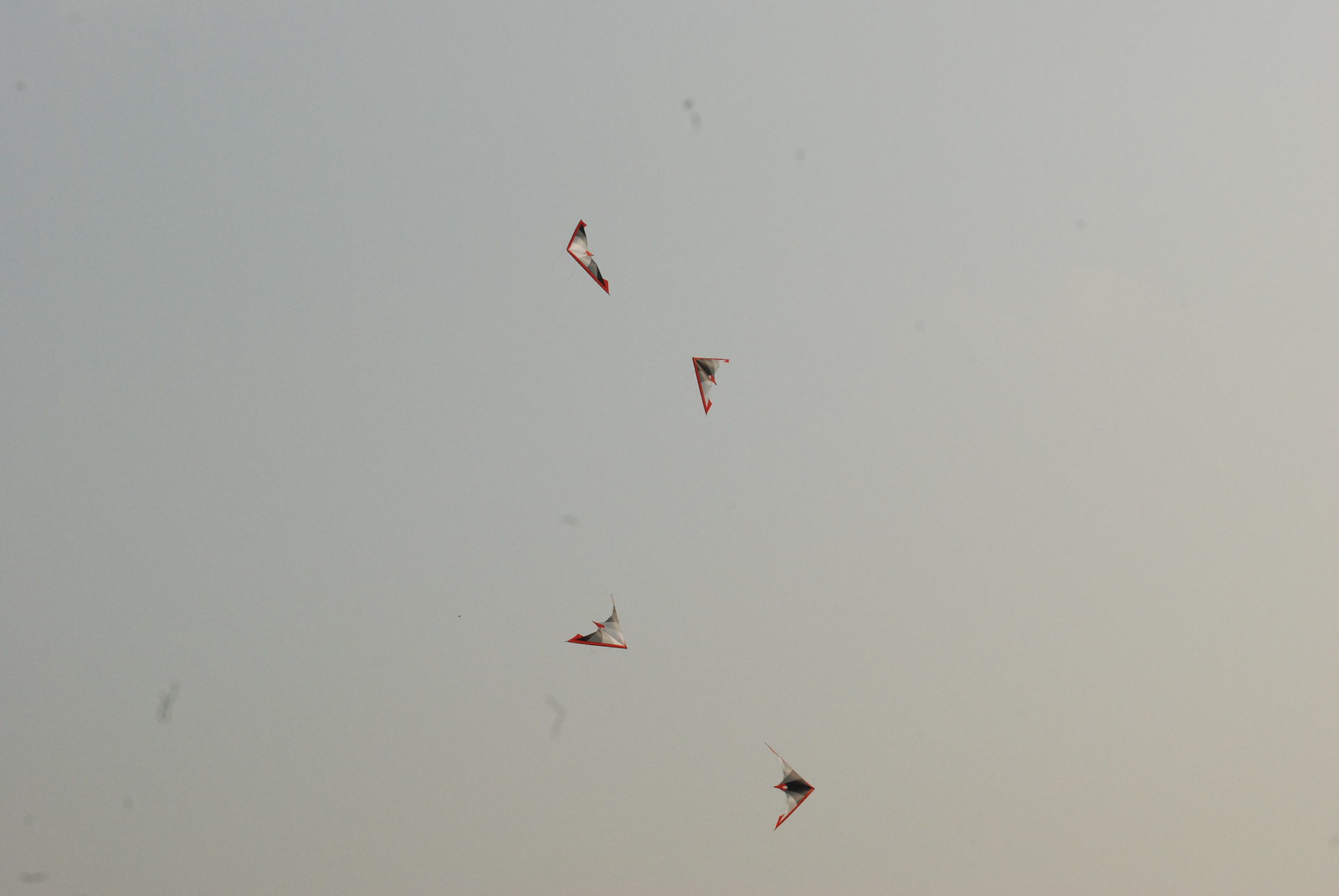The image depicts a vast gray sky, likely overcast and indicative of windy weather with no visible clouds. In this expansive sky, four kites are flying high, their strings presumably invisible due to the distance. These kites have a distinct design: the frame of each is a vibrant red triangle, while the body is white with a black stripe running down the middle. They are oriented in different directions, creating a dynamic scene. Additionally, some indistinct marks, possibly dirt smudges on the photograph, are visible, giving the sky a slightly cluttered appearance.